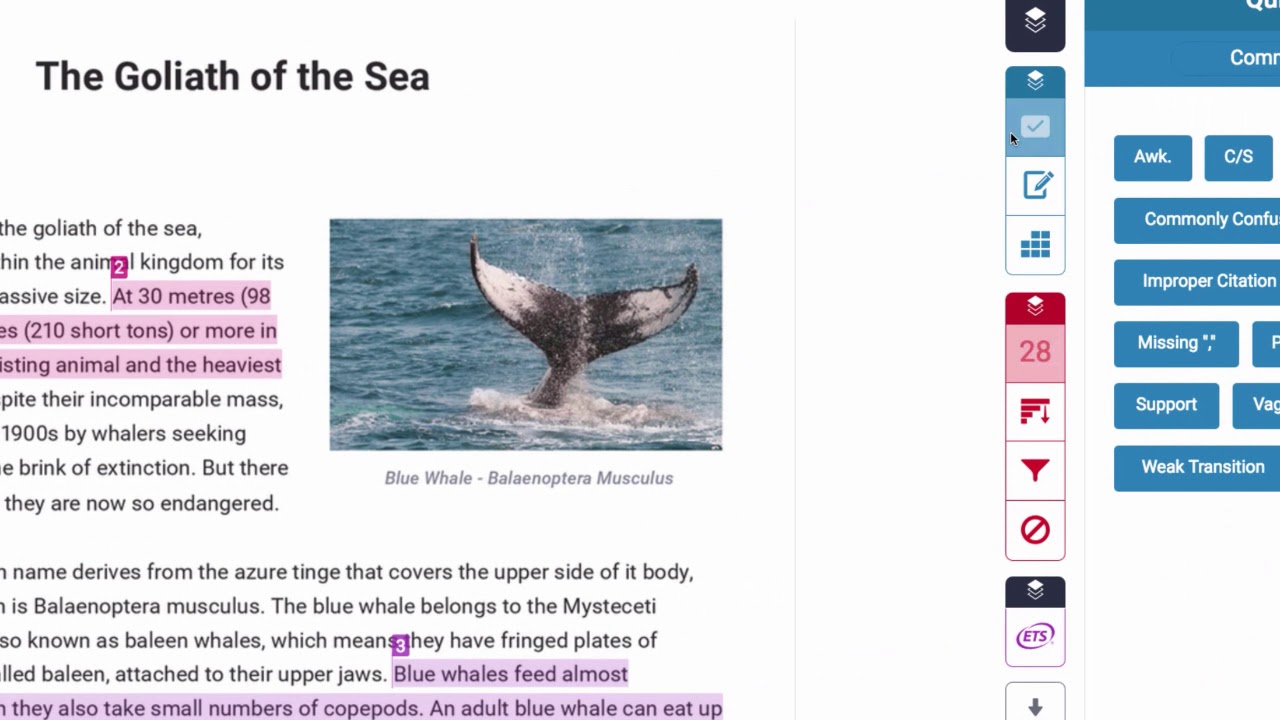In the vast expanse of the ocean, the blue whale, often referred to as the "Goliath of the Sea," reigns supreme in size and presence. Reaching an astounding 30 meters (98 feet) in length and weighing up to 98 tons, its sheer mass overshadows all other marine life. Despite its formidable size, the blue whale is not currently considered to be critically endangered, though it was hunted to the brink of extinction in the past.

The name "blue whale" is derived from the iridescent blue-gray color of its upper side, a characteristic attributed to the tiny organisms known as diatoms that cover its skin. As members of the species Balaenoptera musculus, these magnificent creatures are also classified under the mysticeti suborder, commonly known as baleen whales. This classification indicates that they possess baleen plates in their upper jaws, which they use to filter feed on small prey.

Blue whales primarily consume the smallest lifeforms in the ocean, such as plankton, but they are also known to ingest small quantities of krill and copepods. Astonishingly, an adult blue whale can consume up to 4 tons of krill in a single day.

The image under discussion captures a stunning moment when a blue whale's tail flukes majestically out of the water, contrasting beautifully with the deep blue seascape. This scene might be depicted on an informative website, with additional context provided through tags and buttons on the right side of the webpage, enhancing the educational experience for the viewer.